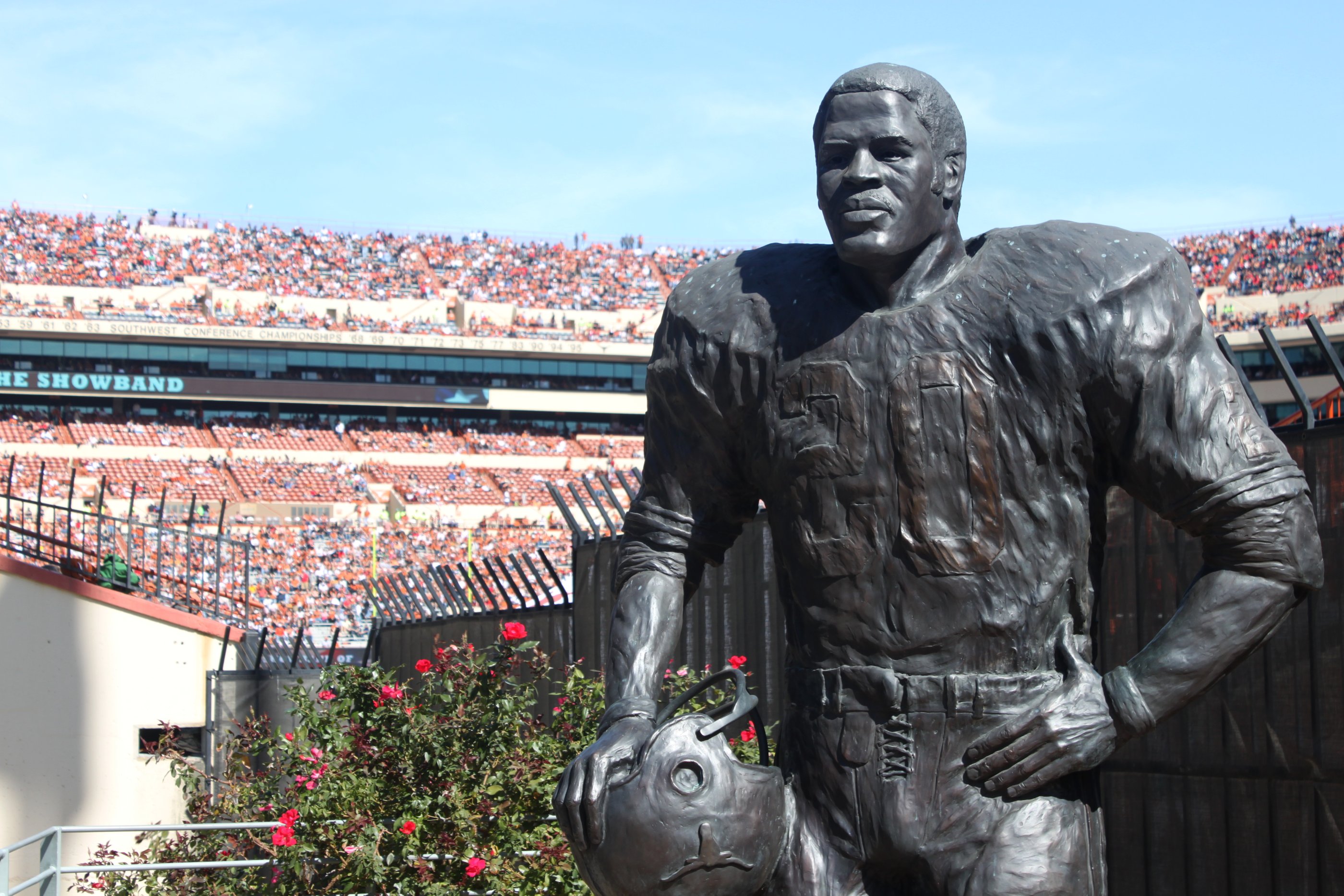This outdoor, daylight photograph captures a detailed image of a statue of a football player situated at a football stadium. The statue, composed of a dark-colored metal, possibly unpolished bronze or black stone, depicts a man with very short hair and set features, wearing a football uniform with prominent shoulder pads. He sports a stern expression on his face and proudly displays the number 20 on his jersey. The football player stands with his left hand on his hip, while his right hand holds a helmet, which features the logo of a bull or steer upside down.

In the foreground, the statue is flanked by a black security fence adorned with spikes to prevent climbing. To the left of the statue, a green bush with vibrant red flowers adds a touch of color. In the distant background, the expansive stadium seating is visible, with rows of orange seats separated into upper and lower tiers, filled with spectators. Above the bustling stadium, a light blue sky with thin, wispy clouds forms the backdrop, completing the scene.